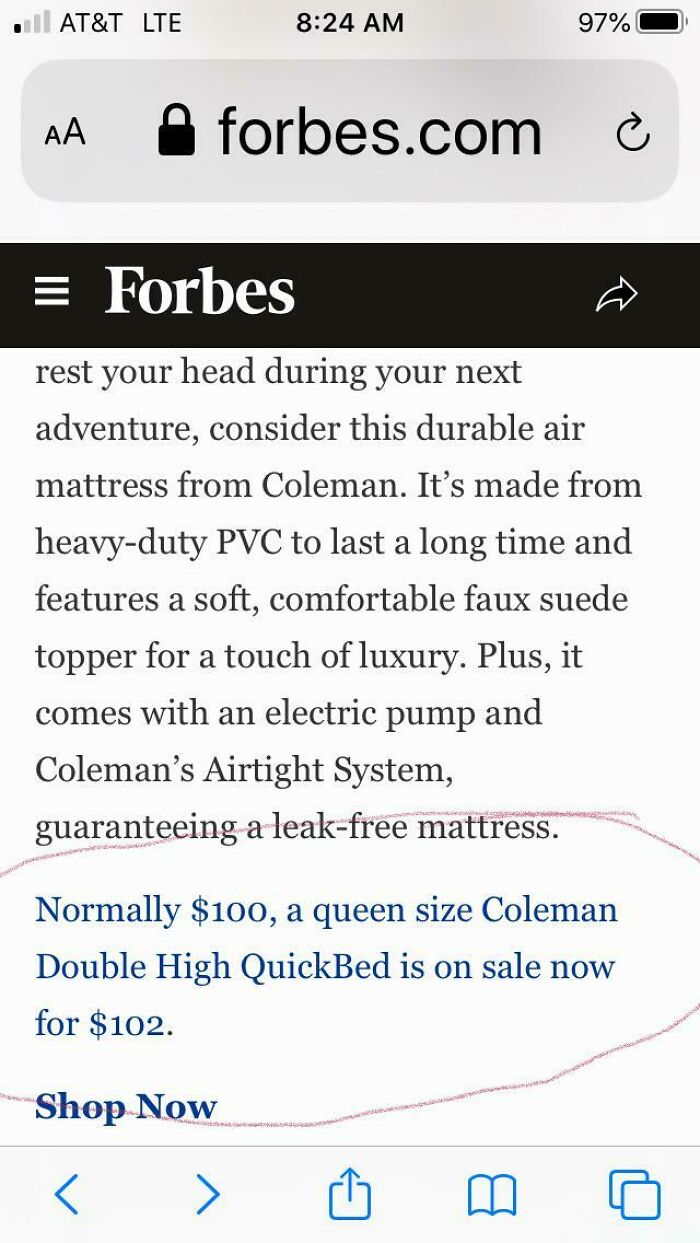The image is a screenshot from a mobile-optimized website. It starts with a grey band at the top, with a gradient effect that is darker in the middle and lighter at the edges, giving the impression of a shadow over the top portion and the box beneath it. 

On the left side of this grey band, there are standard mobile icons indicating signal strength, the carrier "AT&T," and the network type "LTE." In the center, the time is displayed as "8:24 AM," and on the right side, the battery level is shown at "97%."

Below this is a search box displaying "Forbes.com" in large text with a black padlock icon next to it, suggesting a secure connection. Directly underneath, a black bar spans the width of the screen, featuring the Forbes logo in white text. To the left of this logo is a white hamburger menu icon, and to the right, there is a white forward arrow icon.

The main content of the screenshot is on a white background with primarily black text. The text reads: "Rest your head during your next adventure. Consider this durable air mattress from Coleman. It's made from heavy-duty PVC to last a long time and features a soft, comfortable, faux-suede topper for a touch of luxury. Plus, it comes with an electric pump and Coleman's airtight system, guaranteeing no leaks in the mattress."

In blue text underneath, it states: "Normally $100, the queen-size Coleman Double High QuickBed is on sale now for $102. Shop now." 

At the bottom of the screen, there are blue icon buttons for "Back," "Forward," "Upload," "Bookmark," and "Copy." Additionally, there is a red biro marking that circles the blue text about the sale price, possibly highlighting the fact that the item is being sold for $2 more than its usual price, rather than at a discount.